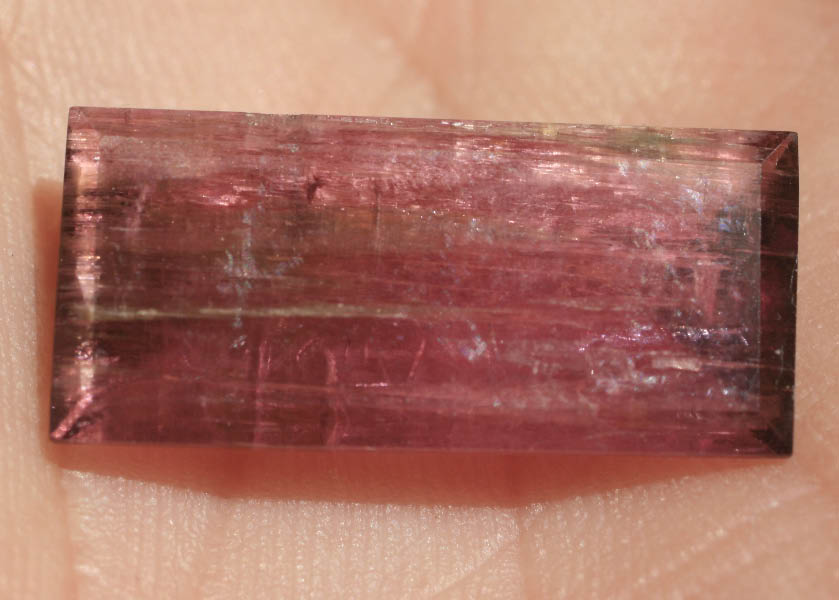The photograph depicts a rectangular, long, red gem with beveled edges, positioned horizontally in the palm of a white person's hand. The hand's creases and lines are clearly visible, accentuating the detailed texture of the tan skin. The gem, streaked with gold and interspersed with dark streaks, notably along the left beveled edge, catches the light, creating visible reflections on some of its facets. The gem appears to be meticulously cut, displaying sharp corners and multiple chips and lines, contributing to its intricate appearance. Although the gem has a predominant pinkish-red hue, there are hints of other colors, including some black on the right edge and a mixture of brown, white, and off-pink among the chips. The image is captured from an overhead perspective, focusing solely on the gem nestled in the palm, with no fingers visible.